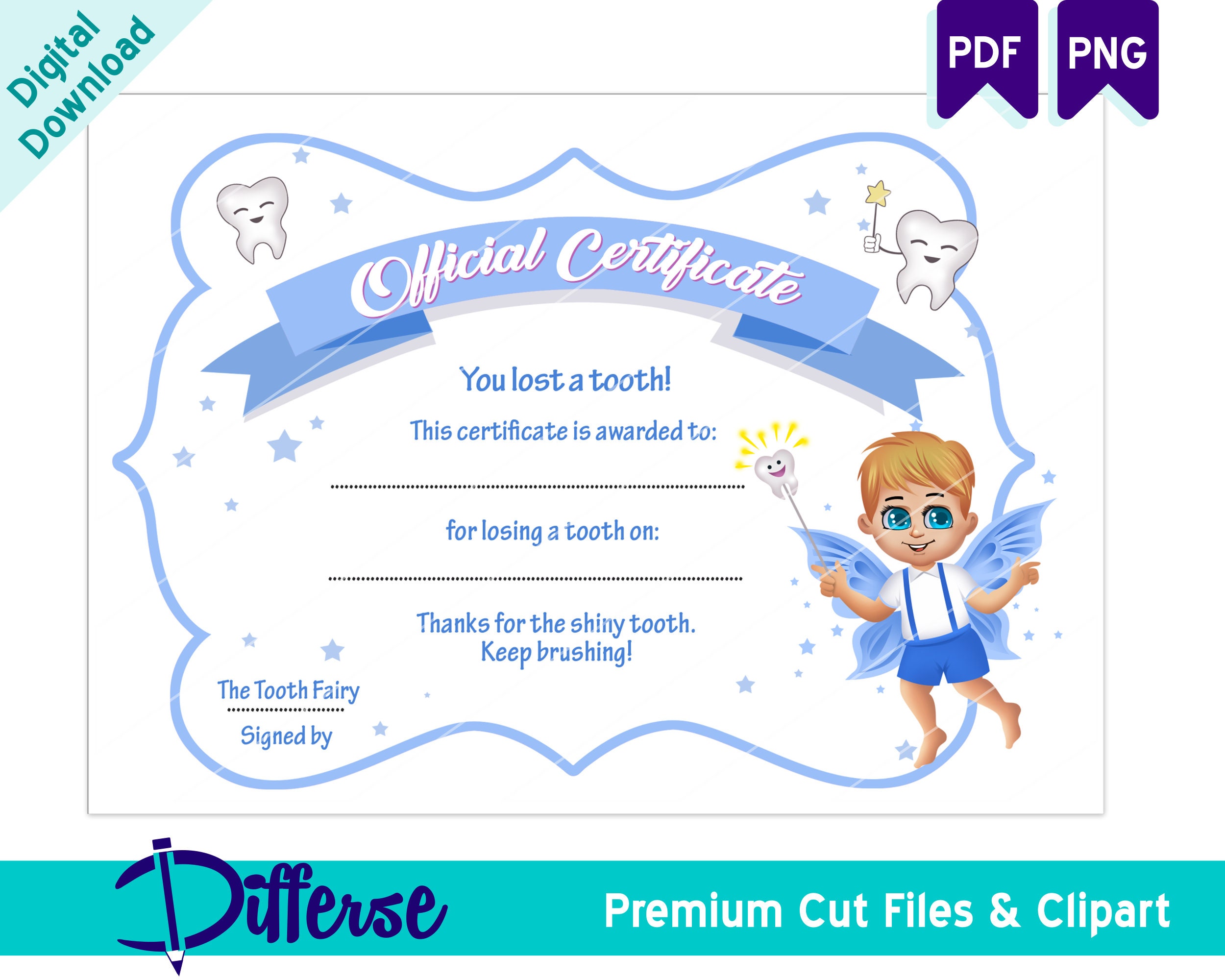This image is of a playful and vibrant digital certificate, designed to celebrate the milestone of losing a tooth. At the top left corner, a green banner reads "digital download," balancing against "PDF PNG" at the top right. The primary design is framed by whimsical, curvy lines and adorned with clip art images of teeth, each featuring expressive faces with eyes and mouths. Prominently, one tooth wields a magic wand topped with a star, adding a magical touch. Centered within the design, a blue ribbon banner states "Official Certificate" in elegant white script. Below, the text celebrates the achievement: "You lost a tooth! This certificate is awarded to..." followed by a blank dotted line for the recipient's name, and another line for the date. A cheerful message reads, "Thanks for the shiny tooth! Keep brushing!" To the right, a charming clip art image depicts a little boy with blonde hair, blue eyes, angelic blue wings, and an adorable outfit of blue shorts and suspenders, complete with a white shirt. He is portrayed as a tooth fairy, holding a wand with a tooth atop it that glows with a golden spark. Finally, a teal banner at the bottom declares "Diffuse" as the brand in bold script, accompanied by "Premium cut files and clip art" in a clean white font.